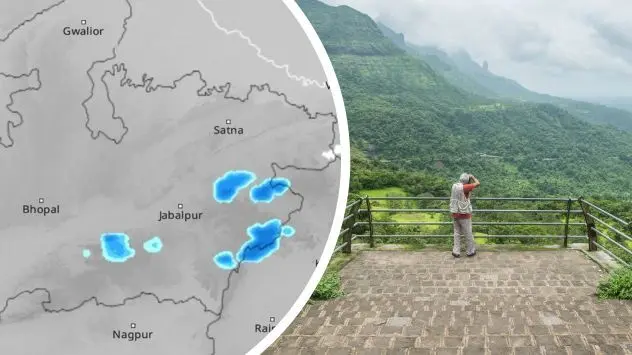The image depicts a striking juxtaposition of a photograph and a graphic overlay. On the right, a photographer stands poised at an overlook with his right hand ready to snap a shot. Dressed in a photographer’s vest, he is positioned at a railing of a fenced observation platform, presenting a secure vantage point over a lush, green, and mountainous rainforest. The landscape is detailed with varied topography, including cloud-covered hills and a verdant, tropical environment. The ground beneath the photographer features a brick pavement.

To the left, a detailed graphic is overlaid on the photograph, displaying an aerial cartographic map of India. The map highlights major city names, boundary lines, and geographical features such as rivers and lakes. Additionally, it displays radar activity indicating cloud cover, giving an impression of ongoing weather conditions. This combination creates a rich, dual-perspective visual showcasing both the natural beauty from the viewpoint and the geographical details of the region on the map.